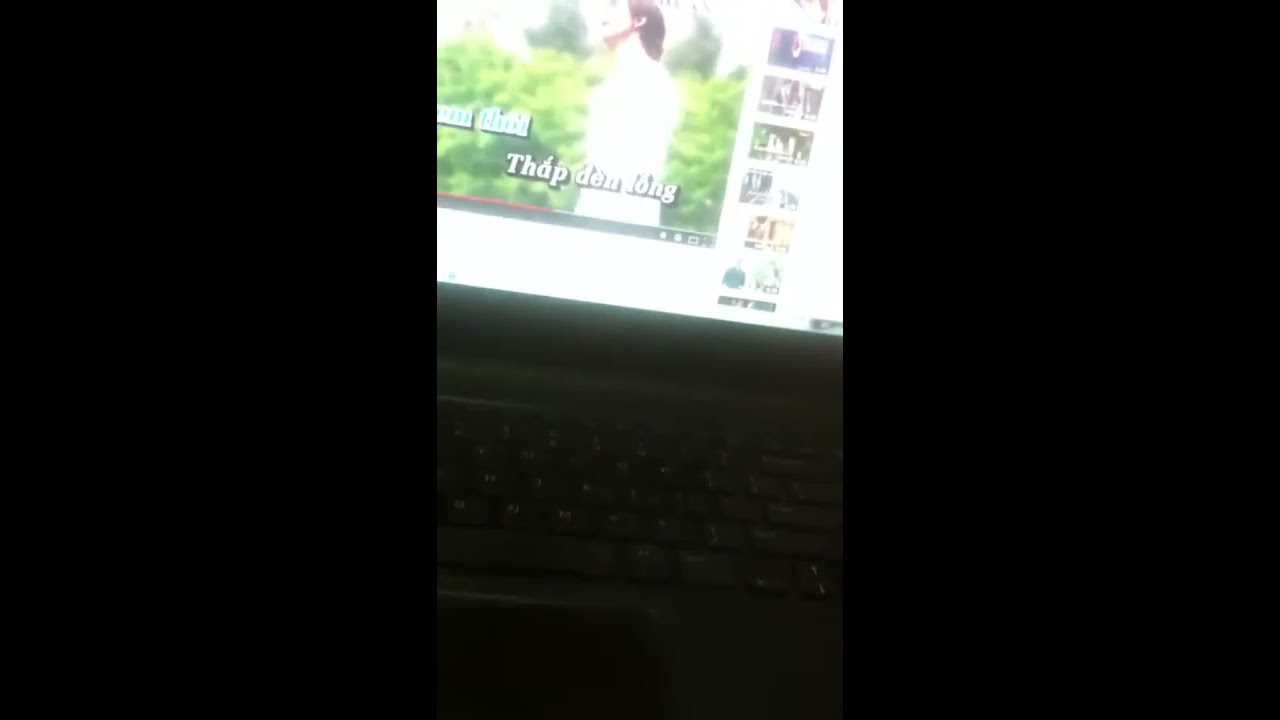This image captures a vertically-oriented, low-quality, and somewhat blurry photograph of a black laptop taken with a cell phone. The scene is very dimly lit, resulting in a lot of black space on either side of the central subject. The bottom portion of the image faintly reveals a backlit keyboard. The laptop screen occupying the top half appears to be displaying a YouTube video featuring a man dressed in white, possibly singing or talking, while standing outdoors, perhaps near a bush. The video includes subtitles that seem to be in either Indonesian or Vietnamese. To the right of the main video, a column of recommended videos is visible.